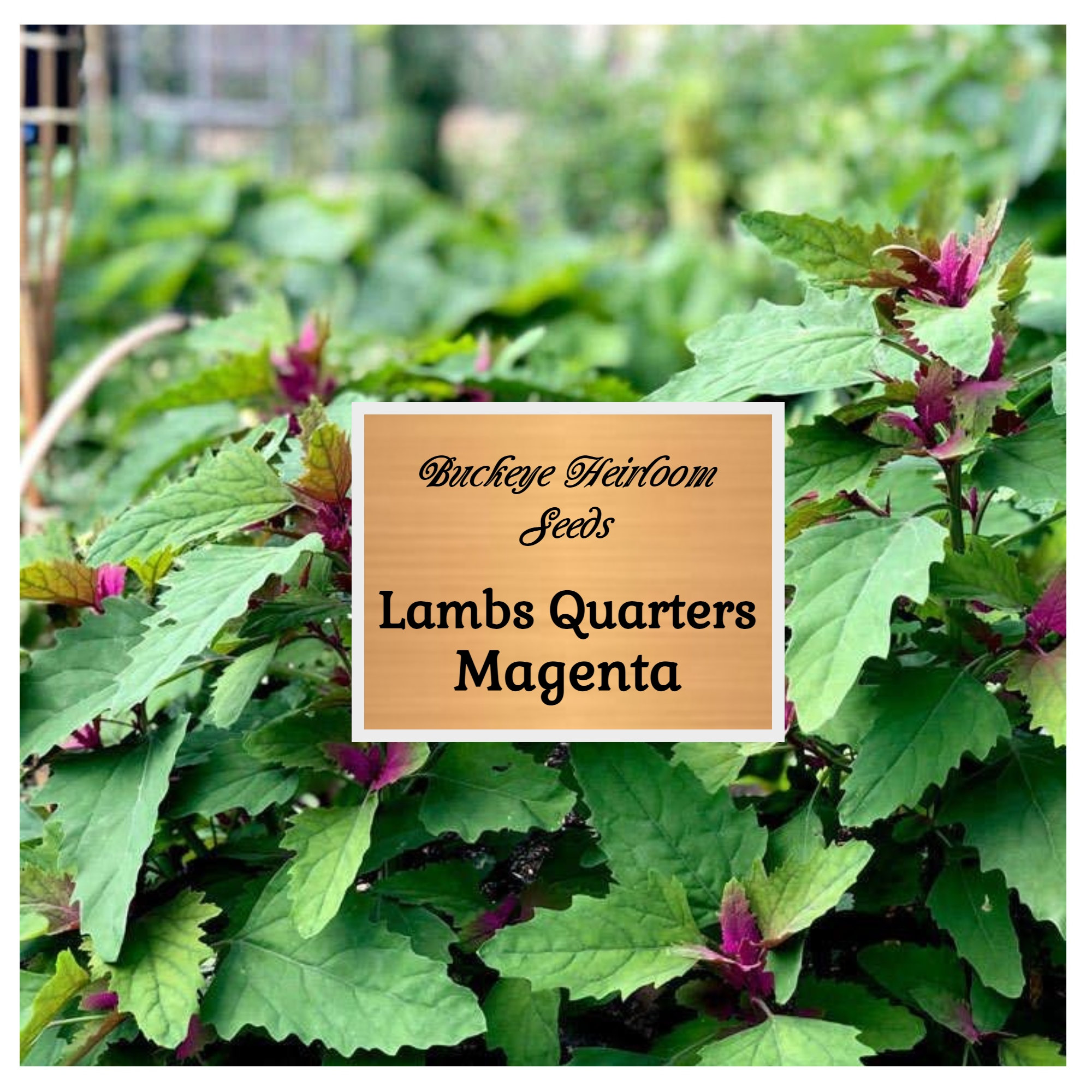This captivating photograph showcases a collection of lush foliage plants. The plants feature serrated green leaves with striking violet-purple undersurfaces. Notably, the emerging leaves at the center of each plant are a vibrant, eye-catching purple. In the background of the image, a tiki torch is positioned on the left side, casting a rustic ambiance, while a gray-painted garden structure stands behind it, adding a subtle, industrial element. The photograph is taken from an up-close perspective, allowing for a detailed view of the foliage, including the intricate veins coursing through the leaves. Central to the image is a square element with a blonde, wood-grained background. This square bears the text "Buckeye Heirloom Seeds" in an elegant black script-style font, and beneath it, "Lambsquarters Magenta" is written in a straightforward black font.